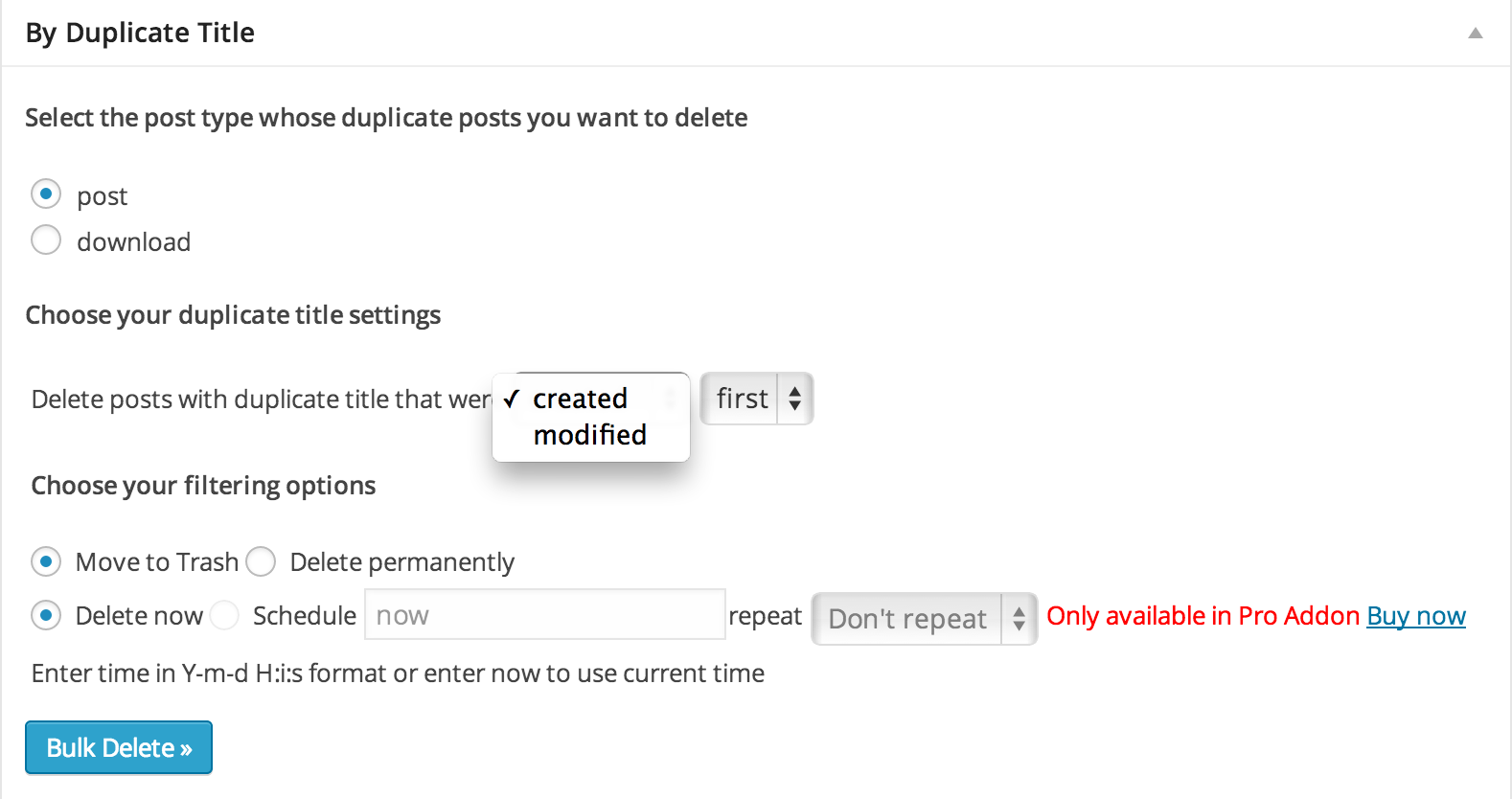This is a detailed screenshot of a website featuring various options for managing duplicate posts. The background of the website is white, and all the text is rendered in black. 

At the top of the webpage, bold black text reads "By Duplicate Title," followed by a thin horizontal line spanning the page's width. Below this, regular black text directs users to "Select the post type whose duplicate post you want to delete."

Underneath this directive, there's a button labeled "Select Post," with "Download Post" currently selected. The next section advises users to "Choose your duplicate title settings." The instruction "Delete posts with duplicate title that were..." is partially obscured by a pop-up. This pop-up is a white rectangle with a check mark, stating "Created/Modified," and the "Created" option is checked. A drop-down menu next to it reads "First."

Further down, the page prompts users to "Choose your filtering options." The choices are:
  - "Move to Trash" (currently selected)
  - "Delete Permanently"
  - "Delete Now" (selected by default)
  - "Schedule"

Following the "Schedule" option, there is an input box for the user to enter scheduling details. The "Repeat" option then appears with the note "Don't repeat." A red note beside it indicates that repeating is "Only available in Pro add-on," followed by a blue "Buy Now" link for users who want to upgrade.

Below these options, there's text instructing users to "Enter time in y-m-d h format or enter now to use current time." 

Finally, in the bottom left corner of the webpage, there's a prominent blue button with white text that reads "Bulk Delete."